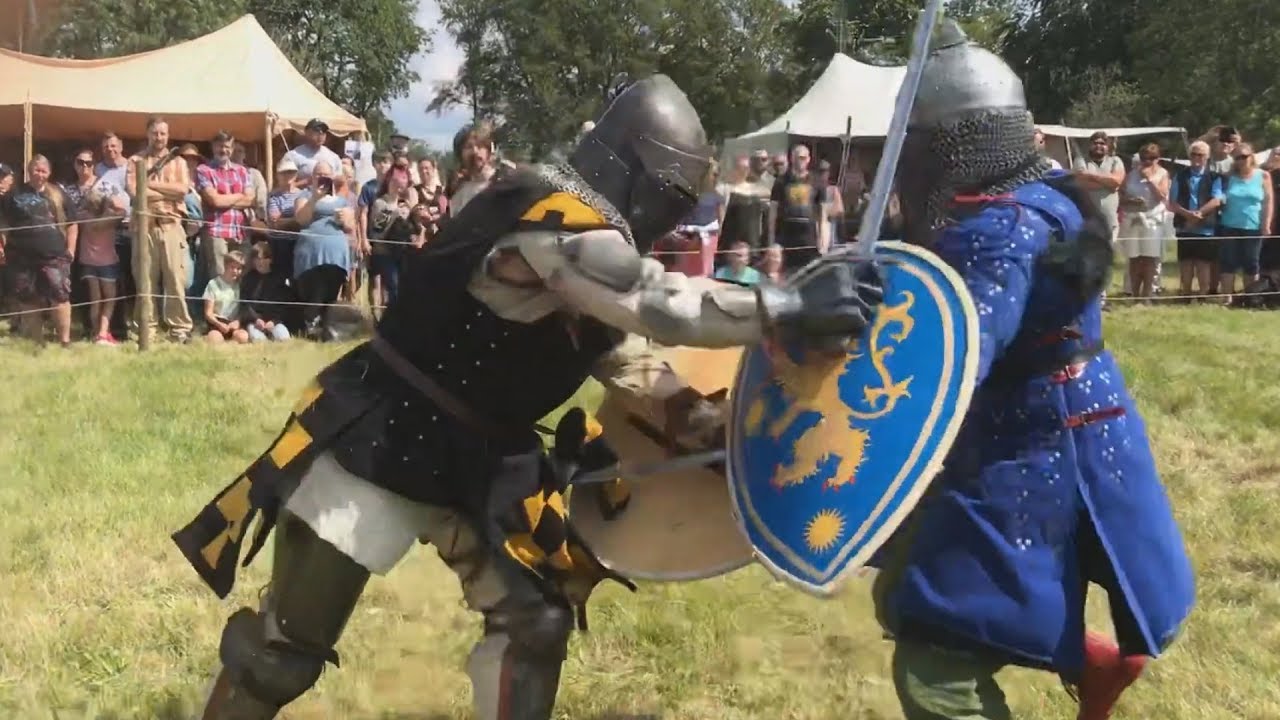In this captivating photograph taken at a renaissance fair, two knights are locked in an intense battle, surrounded by modern-day spectators behind a rope fence. On the left, a bulky knight clad in black and yellow armor with white sleeves and black gloves fiercely pushes against his opponent's shield. His black helmet and chainmail provide a stark contrast to the vivid yellow and black cloth draped over his attire. With a sword in his right hand and a shield in his left, the black knight's powerful stance is evident as he tries to overpower his foe. To the right, a knight adorned in blue with a silver helmet and chainmail, and a ponytail visible, is equally determined. He wields a blue and yellow shield and appears to be maneuvering his sword toward the black knight's thigh in a strategic strike. The grassy field setting, along with the colorful tents and trees in the background, enhances the historic ambiance, while the blurred action of the jousting knights adds a dynamic energy to the scene.